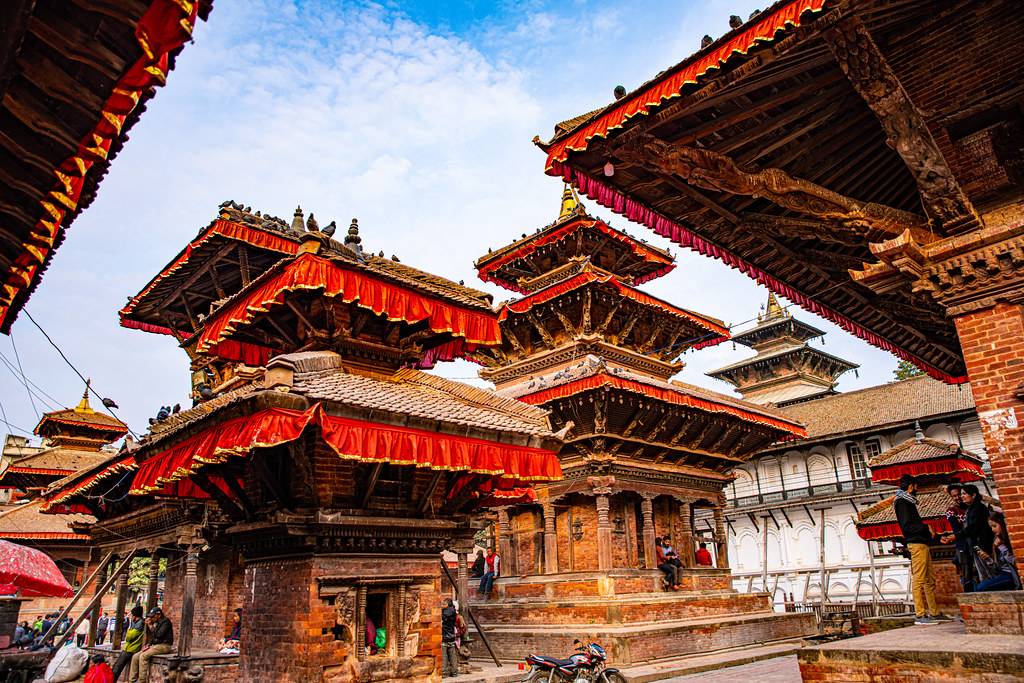This photograph features a set of traditional Asian temple-like structures, captured outdoors during the daytime under a sky mostly filled with white clouds and a hint of blue at the top center. The buildings are characterized by tiered, square bases made of red brick, ascending with smaller, tiered roofs adorned with dark tiles. Each tiered section of the roof has red drapes with gold edging hanging down from the eaves. The buildings are primarily three-tiered, with the one on the left being shorter but still having three layers, and the one on the right being taller with three layers as well. In addition to the main structures, there is a less distinct white building in the background. The area is populated with people; some are seated on the brick steps, while others are standing around, conversing and observing the architecture. The intricate design and the tiered arrangement of the buildings evoke a traditional Asian aesthetic, highlighting an atmosphere reminiscent of historical temples.